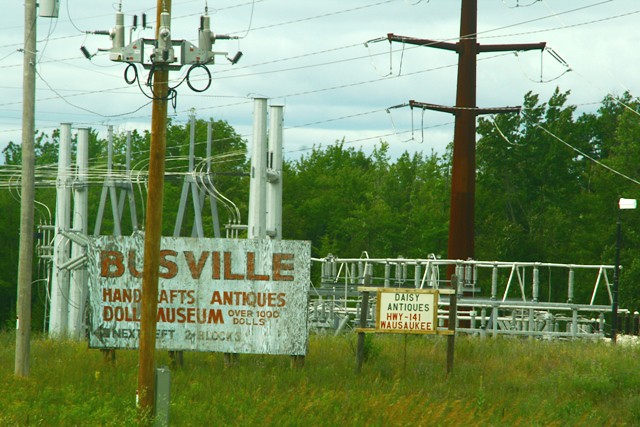The photograph, taken outdoors, captures a tangled web of power lines and assorted cables crisscrossing the frame. The upper portion of the image features a mostly cloudy sky, rendered in overcast, stretched clouds that give the sky a pale, almost whitish hue with hints of blue peeking through. Below the sky, a row of dark green trees lines the horizon, their varying heights creating a subtle visual contrast amidst the landscape.

Dominating the midsection of the image, numerous power lines of differing colors—dark brown, gray, tan—crisscross and stretch across the scene, contributing to an intricate network of infrastructure. Amongst this maze of wires, an old, gray sign with weathered white and gray streaks can be seen. Adorned in red bubble letters, the sign reads "Bustville." A partially obstructing pole hides some of the text, but the visible portion hints at an advertisement for "Handcrafts Antiques Doll Museum," boasting over a thousand dolls and indicating directions to the next left. Below, a smaller sign directs drivers to "Daisy Antiques on Highway 141, Wasaki."